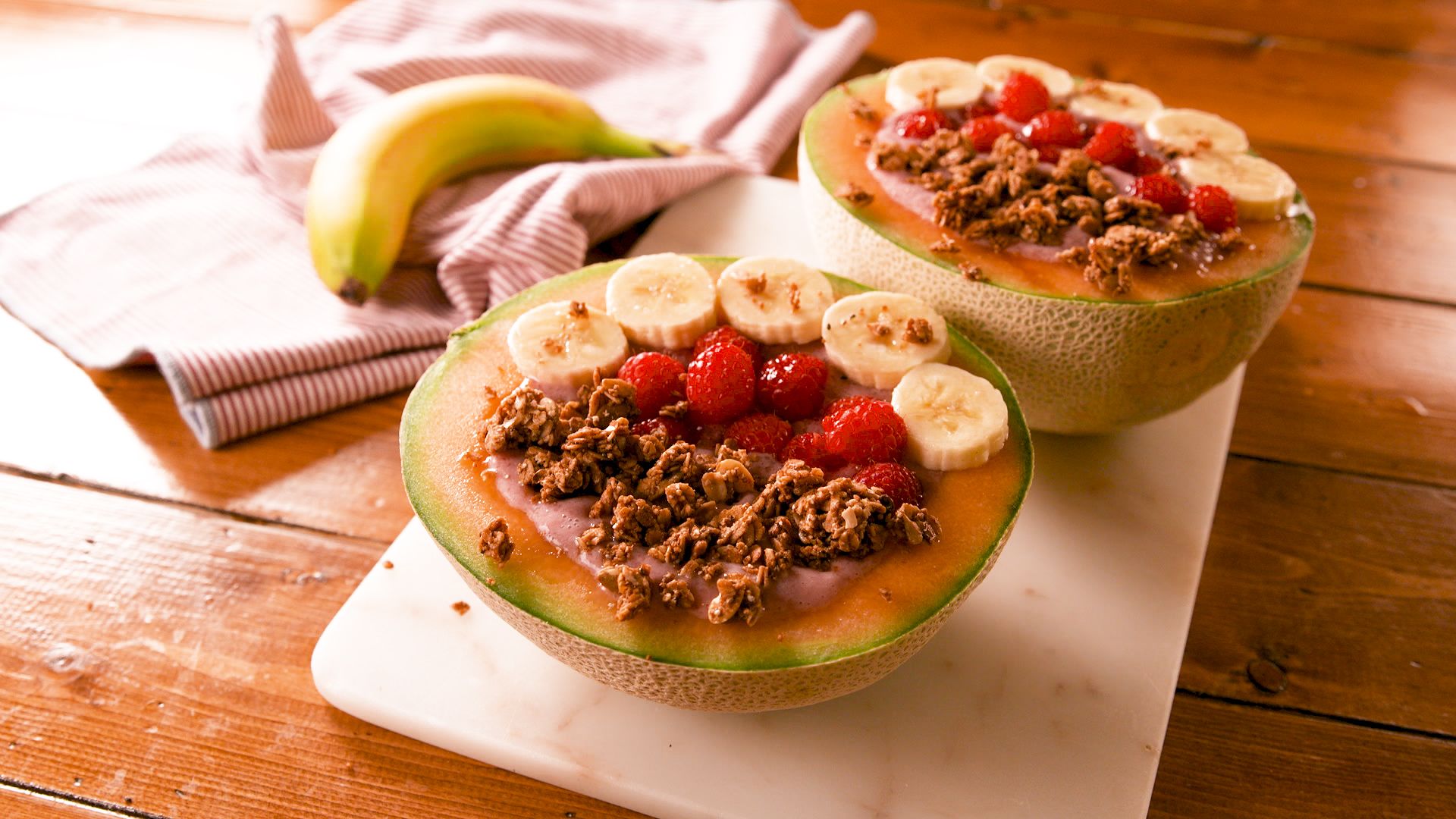In this photograph, two cantaloupes have been halved and placed side by side on a white marble cutting board featuring beige flecks. The cutting board rests on a lightly stained, roughly hewn wooden table with visible grain patterns. The cantaloupe halves are artfully filled, creating a vibrant cantaloupe fruit bowl presentation. Inside each hollow, a base of pink yogurt is nestled beneath layers of granola, raspberries, and carefully arranged banana slices forming an arch. Toward the upper left of the composition, a slightly crumpled white fabric napkin with pink stripes can be seen, on top of which lies a not-quite-ripe banana, displaying hints of green at its ends. The scene is well lit, with light entering from the left, illuminating the various textures and colors to create a fresh and inviting presentation.